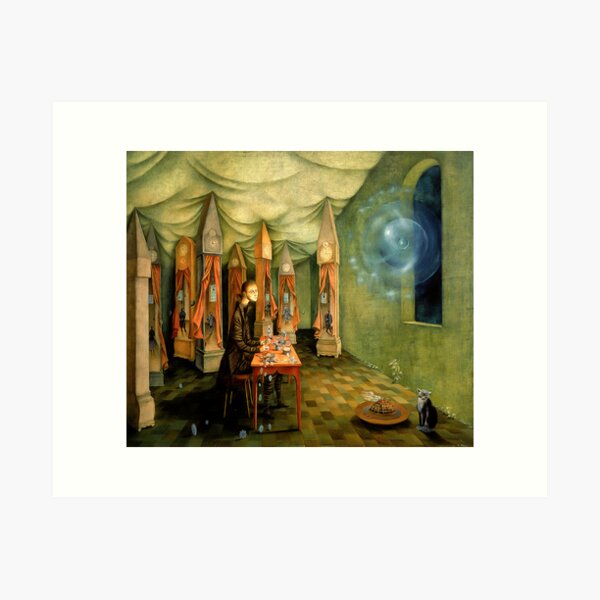The artwork "Revelation the Watch" by Varro is a surrealist color painting set in a medieval-style interior. Dominating the scene is a man, dressed in a long black gown with his hair pulled back, seated at an orange rectangular table to the bottom left of the image. He gazes up at a ghostly, bluish and translucent spherical object that appears to be mystically entering or exiting through an arched window on the right side of the room.

The room itself is vividly detailed: the green walls are adorned with tall, brown wall clocks that have pointed tops resembling pencils. These clocks are partially concealed by orange curtains pulled back to reveal small figures within. Above, the ceiling is draped with white and greenish fabric, creating an uneven, pillow-like texture that mimics a tent.

The floor is made up of brick-shaped tiles in a checkerboard pattern of earthy colors—browns, whites, and greens—adding to the grounded, historical feel of the space. In the lower right corner, a cat sits on its hind legs beside a brown food dish, completing this enigmatic scene. The overall color palette includes orange, white, brown, green, and grayish blue, enhancing the surreal yet historical ambiance of the painting.